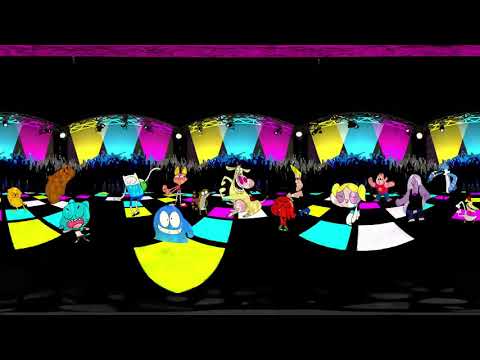In this vibrant and dynamic animated scene, a variety of colorful characters take center stage against a detailed and engaging backdrop. Central to the composition is a unique character dressed in a blue outfit, distinguished by having eyes and a mouth on its body. This figure stands prominently on a distorted yellow square, which itself lies on an elaborately patterned checkerboard floor in black, yellow, aqua, and magenta hues.

Behind this central character, the scene unfolds with a teal square and a darker pink wall, creating depth and contrast. Adjacent to the blue character are numerous imaginative creatures: to the immediate left, a cat-like figure with extraordinarily long arms and yellow ears; to the right, a cow character with its mouth agape, donned in a yellow suit. Nearby, a lady in a black coat holds a red dress, adding further intrigue to the ensemble.

The scene is enriched with decorative banners hanging from the top. These banners, designed as downward-pointing triangles, exhibit a vibrant color palette of yellow, teal, and purple, repeated in five sets across the stage. Above the banners, a purple bar stretches horizontally, bordered by a black bar at the very top, all set against a predominantly black background.

This animated image pulsates with action and color, capturing a festive atmosphere where various cartoon characters, resembling ghosts, mice, and whimsical figures in blue, red, and pink with yellow hair, appear to be dancing and enjoying the lively scene.